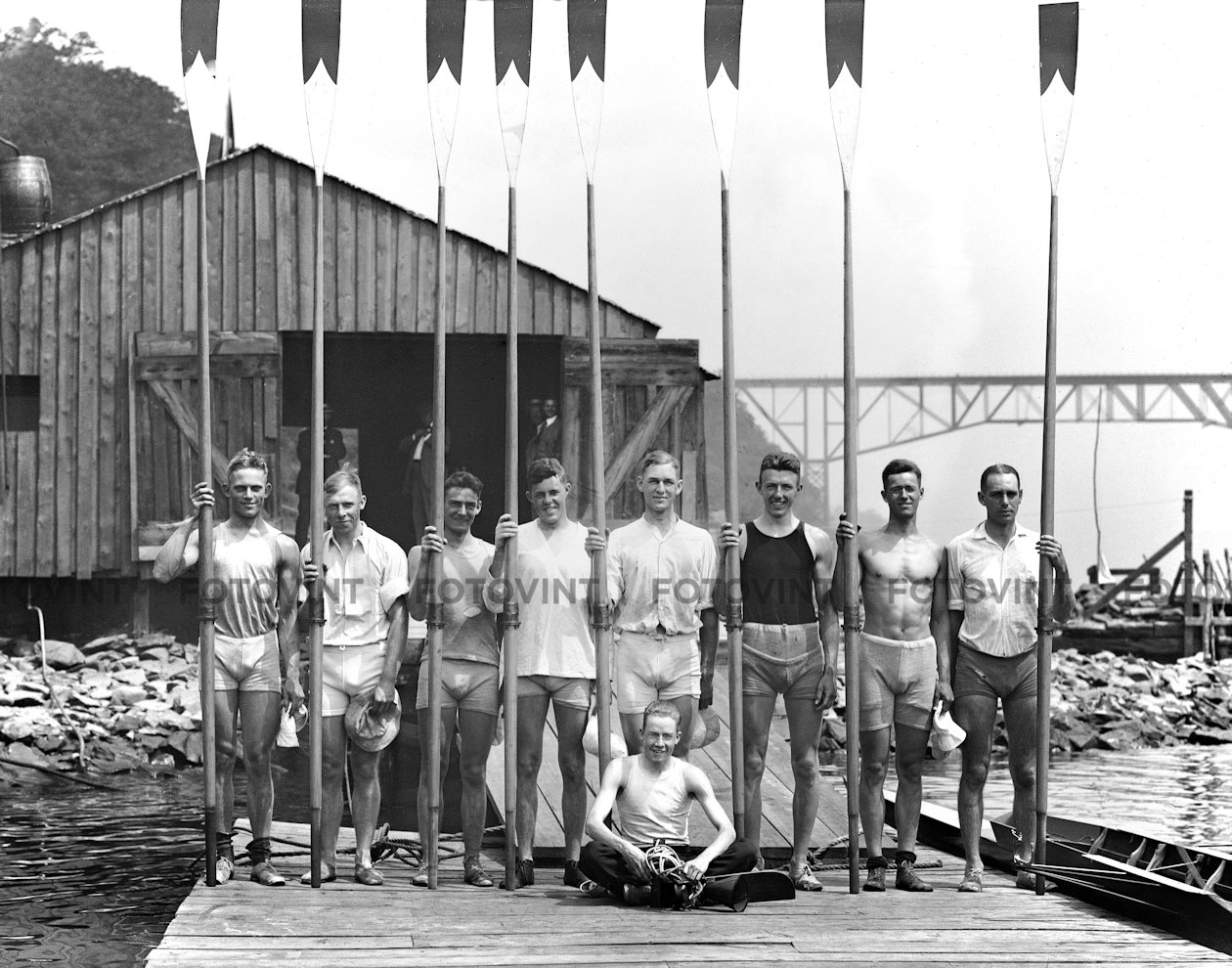This black and white vintage photograph captures a rowing team standing on a dock, exuding a timeless and classic vibe. The team consists of eight rowers and their captain, making a total of nine individuals. Each rower is holding a rowing oar, towering over them at twice their height. The rowers are dressed mostly in white shirts and shorts, with one member distinguishable by a black vest. The captain is seated in the front, presumably orchestrating the team. Behind the team, a wooden warehouse stands with other gentlemen in suits observing the scene from inside. The right side of the photograph reveals an element of old-world chaos with a metal bridge (likely a railway) and assorted wooden and metal parts scattered along the riverbank. The image captures an outdoor setting in the daytime, devoid of any text, encapsulating a moment of sporting camaraderie against a backdrop of industrial scenery.